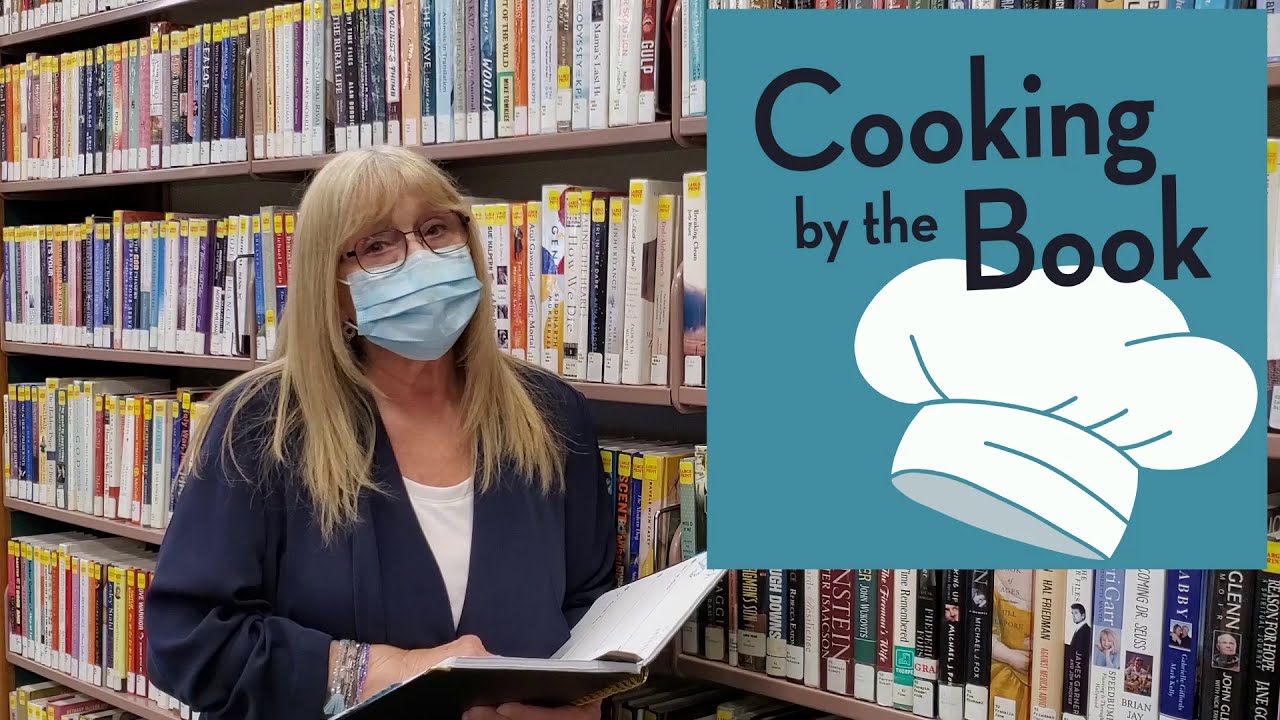In this detailed photograph, a blonde-haired Caucasian woman stands in a library, surrounded by rows of books shelved neatly behind her, all labeled with yellow Dewey Decimal symbols. She is attired in a navy blue blazer over a white t-shirt, her light blonde-brown hair cascading past her armpits and accentuating her look with wire-rimmed glasses and a blue surgical mask. Her right wrist adorned with bracelets, she has her head tilted to the right in a thoughtful pose while holding an open book at waist level, supported by her bent elbow and left hand. The image is in landscape orientation, with a distinct overlay on the right side: a teal blue rectangle featuring the text "Cooking by the Book" in black letters, accompanied by an icon of a white chef's hat. The promotional rectangle partially obscures the scene of the library, inviting viewers to engage with the picturesque setting and the intriguing title in tandem.